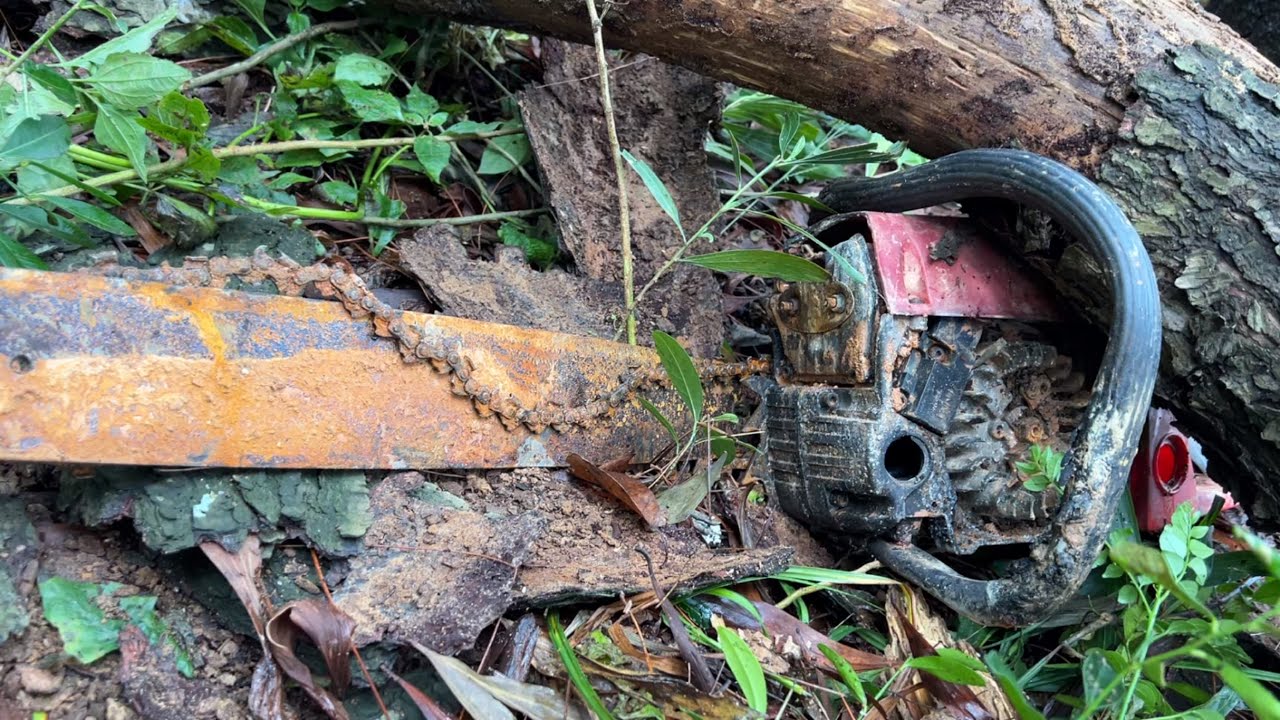This color photograph depicts a decrepit and abandoned chainsaw lying on the ground in a wooded area, surrounded by fallen leaves and dirt. The chainsaw's motor, housing, and black handle are visible on the right side, appearing dirty and weathered, with the gas tank top missing and exposing just a black hole. The rusty blade extends to the left, with the chain having come off and laying haphazardly on top of the blade. The scene is further characterized by the presence of a large, rotting tree trunk with grey bark and brown wood, which appears to have fallen, possibly trapping the chainsaw underneath. The trunk stretches diagonally from the middle right to the top of the image. The surrounding area is cluttered with scattered pieces of wood, grass, weeds, and additional vegetation, suggesting that the chainsaw has been abandoned for a considerable amount of time.